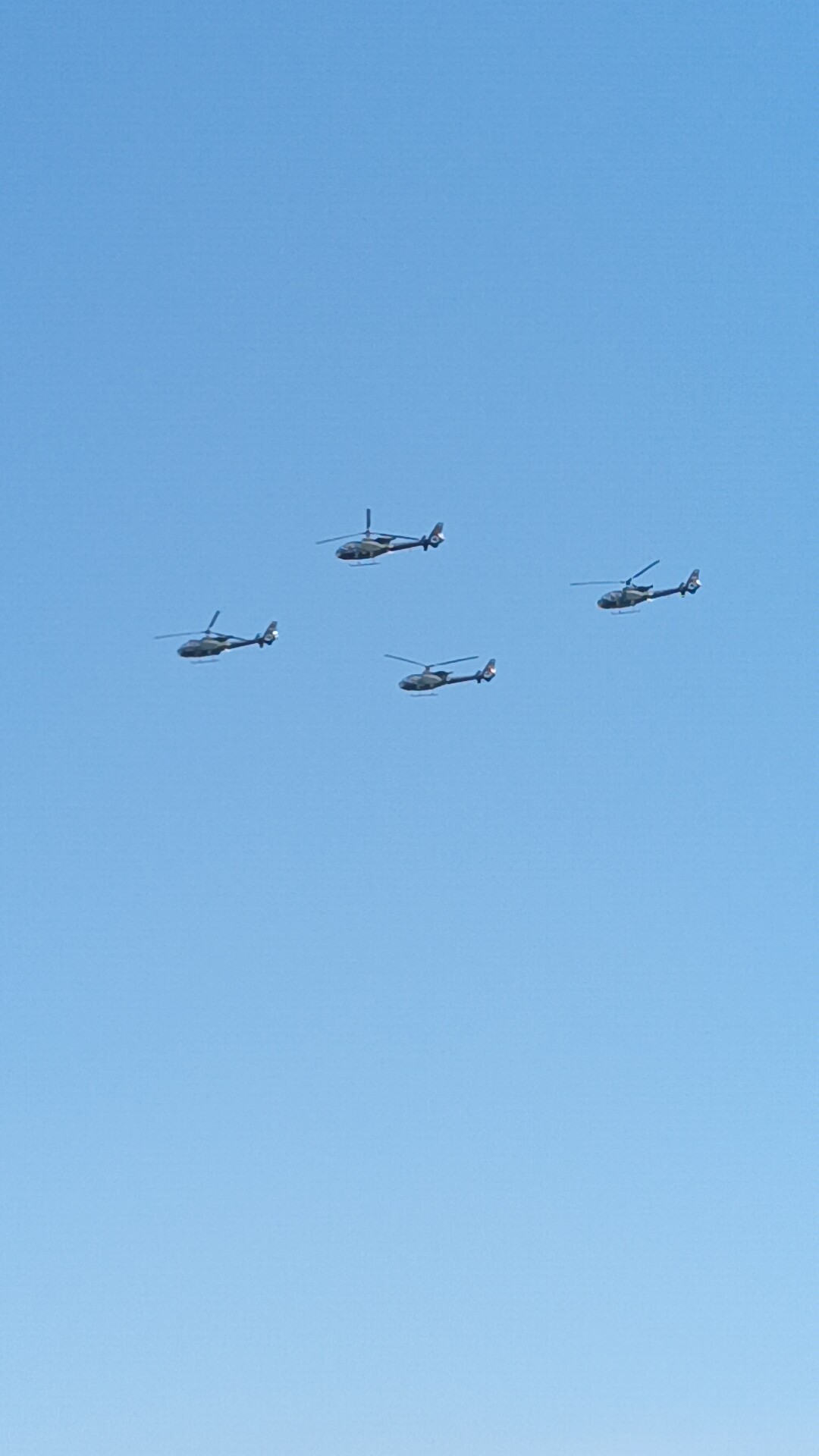This captivating photograph captures a vast, clear blue sky with a subtle gradient, transitioning from a darker blue at the top to a near-white at the bottom. Taken from the ground with the camera pointed directly upwards, the image is devoid of any surrounding environment, focusing solely on the sky itself. Prominently featured in the center of the frame are four dark gray helicopters flying in a precise formation, resembling either a diamond or square shape. The helicopters appear slender and narrow, differing from the bulky profile typical of military aircraft, with each displaying three-bladed propellers. The farthest left helicopter leads the group, followed by two helicopters vertically aligned above and below it, and a fourth one trailing behind in line with the leader. The helicopters seem small against the expanse of the sky, indicating their significant altitude. With no clouds or birds to distract, the serene, unblemished blue sky highlights the striking, synchronized flight of the helicopters, possibly suggesting a formation flight or aerial show.